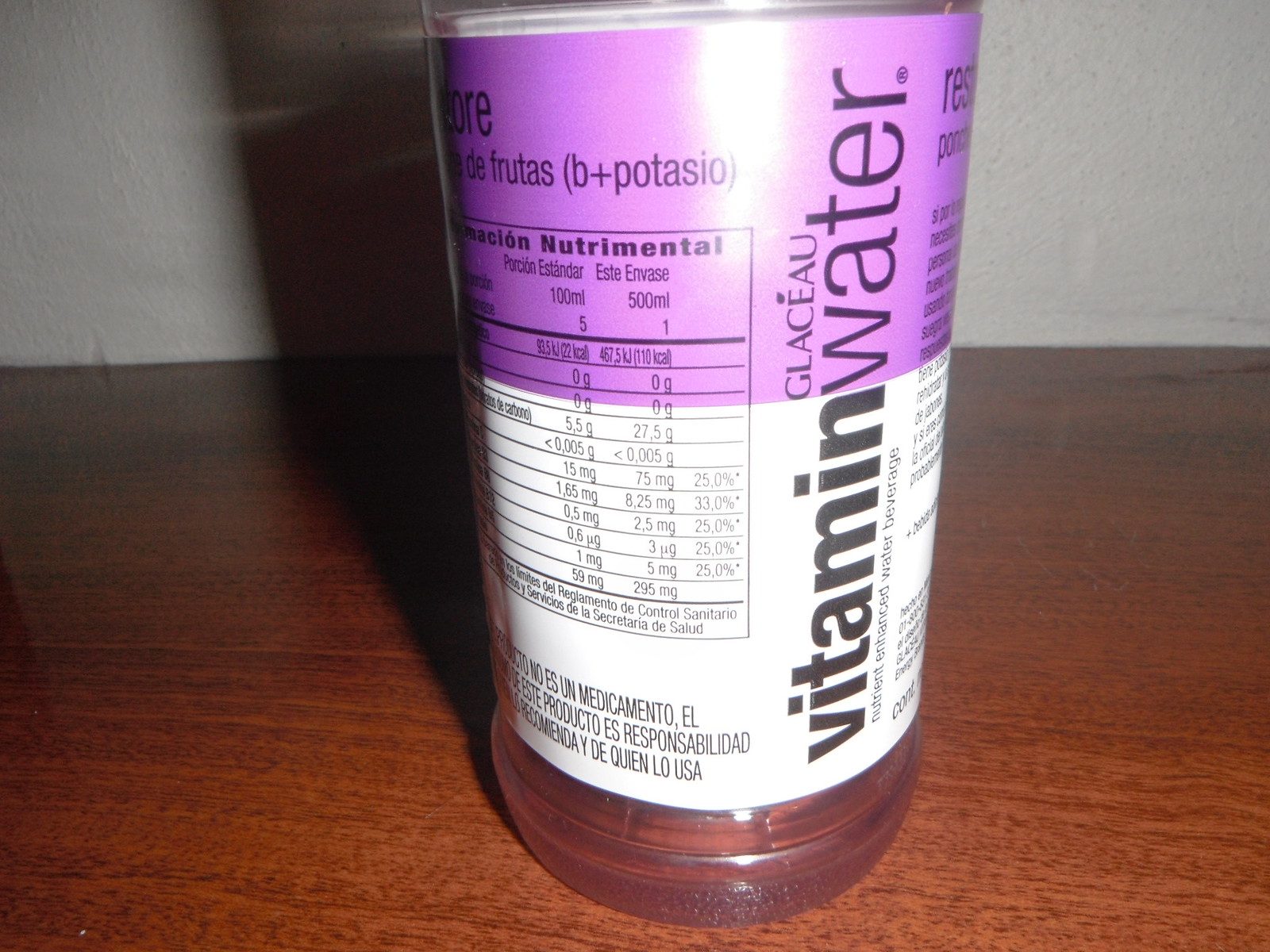This detailed photograph captures the lower half of a clear plastic bottle of Vitamin Water, prominently featuring a distinct purple and white label. The bottle is positioned on a dark brown faux wood table, which is set against a stark white wall. At the bottom of the bottle, visible through the clear plastic, is a small amount of purple liquid. The label displays "Vitamin Water" in a vertically arranged font with the "V" starting at the bottom and the "R" ending near the top. The upper half of the label is purple, reading parts of the text "O-R-E" and "de frutas B plus potassio," hinting at a potassium-enriched drink. The lower half of the label is white, containing nutritional information in Spanish and possibly details about the product's origin, with words like "nutrimental" and “producto, es responsabilidado.” The photograph appears to have been taken with a flash, as indicated by the reflection on the label and the sharp shadow cast by the bottle onto the table and white wall behind it.